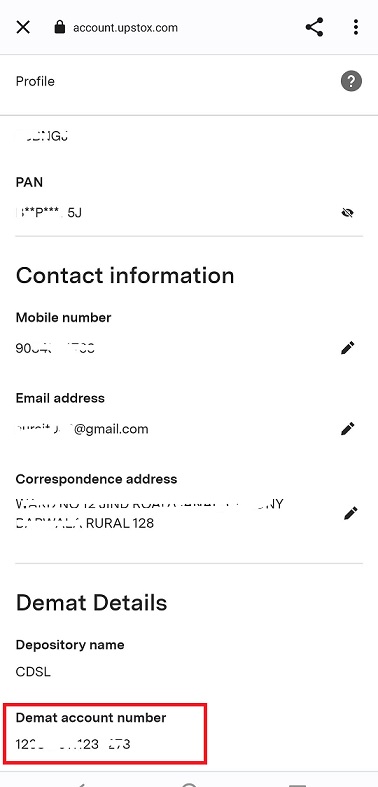Screenshot of a mobile browser displaying the profile page on account.upstox.com. The header of the page features a dark gray circular icon with a white question mark, resembling a help button. The profile information includes categories such as "PAN" with sensitive details obscured by asterisks and a crossed-out eye icon indicating hidden information. The "Contact Information" section lists fields like "Mobile Number", "Email Address", and "Correspondence Address", with the email partially visible, ending in "gmail.com" and the address concluding with "rural 128". Further down, the "DMAT Details" section reveals "Depository Name: CDSL" and a concealed "DMAT Account Number". All critical personal details are deliberately crossed out in white strokes to protect privacy.